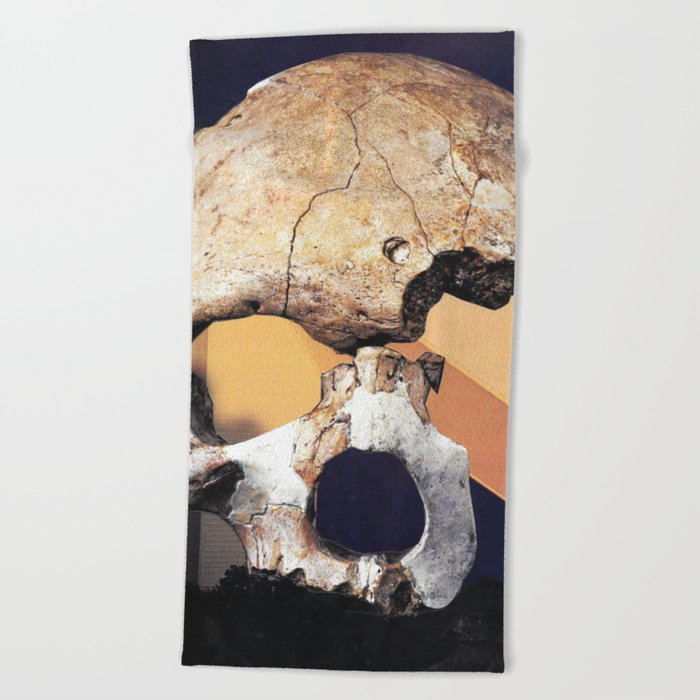The photograph captures an ancient tapestry depicting a deteriorated human skull. The skull, which shows significant signs of aging, is an off-white color interspersed with brown patches, indicative of both time and environmental wear. The skull is positioned to face the viewer directly, although the entire left half (from the viewer's perspective, the right side) is missing, accentuating its decrepit state. The eye sockets of the skull are faintly visible, adding to its macabre appearance. The background of the tapestry is ambiguous but appears to be a wall with varying shades of beige and brown, intersected by a prominent brown stripe and accented by patches of black. The tapestry is not mounted on a rigid frame and is displayed on a white wall, further highlighting its delicate and aged nature.